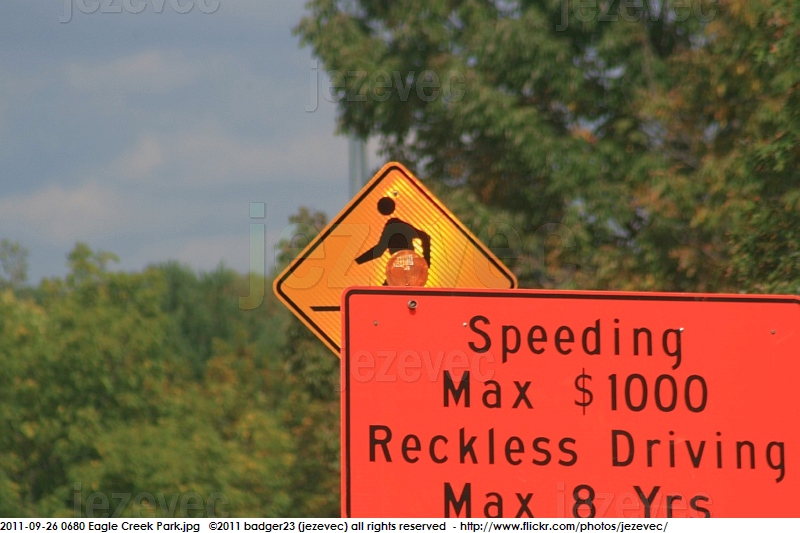In this image, a vibrant blue sky with scattered clouds serves as the backdrop, contrasting against the lush, green leafy trees that show early signs of autumn browning. Dominating the foreground is an orange rectangular sign with black borders, stating in bold black letters: "Speeding max $1,000, reckless driving max 8 years." Positioned near it is another sign, either orange or yellow (difficult to ascertain due to the glare from the sunlight), indicating a crosswalk. This second sign might lean towards orange, aligning with the construction theme of the first sign. Further into the center of the frame, a cell phone tower extends upwards, though its peak is obscured by the surrounding trees. The composition captures the interplay between man-made structures and the serene natural environment.